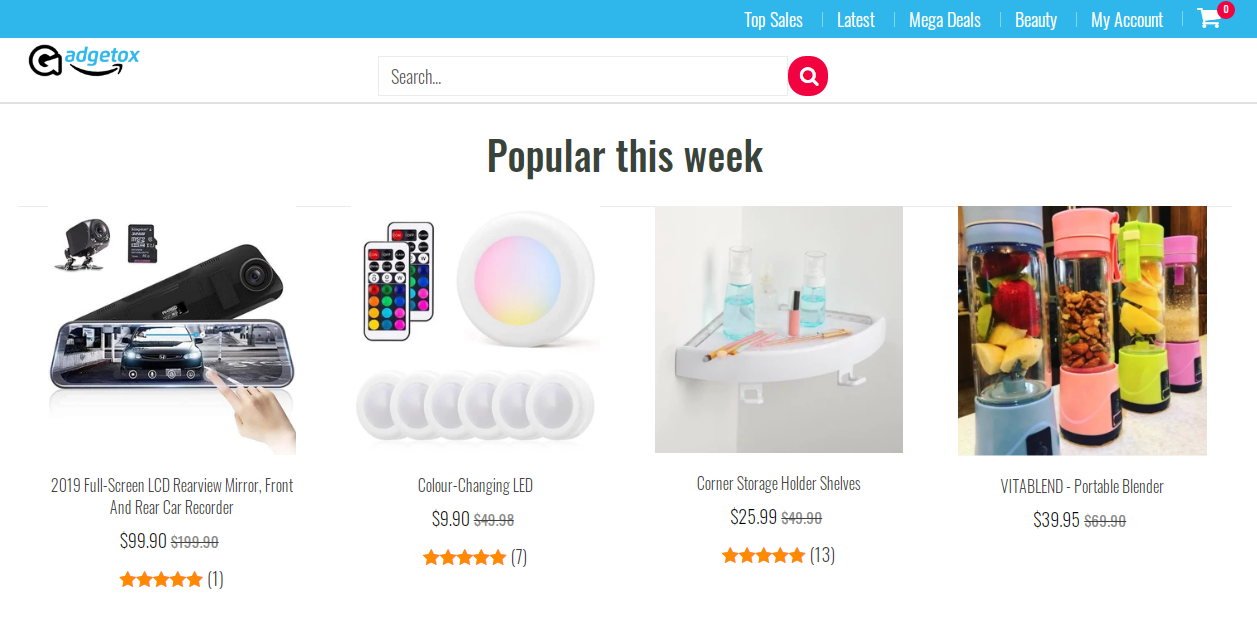This screen capture from a shopping website highlights various sections and products available for purchase. At the top, a blue navigation bar displays categories: Top Sales, Latest, Mega Deals, Beauty, My Account, and an indicator that there are five items in the Shopping Cart.

Below the navigation bar, the website's name, "G Gadget Talks," is prominently featured with a stylish swoop and arrow design. Adjacent to this is a search bar with the placeholder text "Search..." and a red notification bubble.

The main section begins with the heading "Popular This Week," showcasing several featured products. 
1. A 2019 Full Screen LCD Rear View Mirror Front and Rear Car Recorder is displayed, priced at $99.90.
2. A color-changing LED light is illustrated.
3. A Corner Storage Holder Shelf for showers.
4. A Vitablend Portable Blender is shown in multiple colors, priced at $39.95.

Overall, the screen capture encapsulates the layout and offerings of a typical online shopping website, emphasizing various electronics and home accessories.